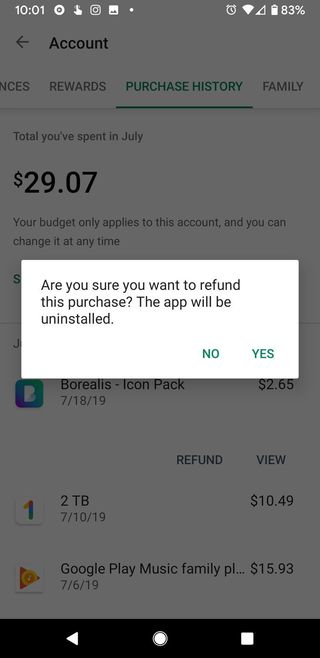The image captures a screenshot of an Android phone's display, featuring both the notification bar at the top and the navigation bar at the bottom. At the top left, various status icons are shown, including an 83% battery level, low cellular reception, an alarm icon, and a full Wi-Fi signal. There are also five notification icons visible.

The center of the screen is dominated by a pop-up message from the Google Play Store, asking, "Are you sure you want to refund this purchase? The app will be uninstalled." This pop-up includes two clickable options: a green 'No' and 'Yes' text.

Behind the pop-up, the screen shows the Google Play Store's account section, slightly grayed out. Visible headings include 'Account,' with tabs for 'Rewards,' 'Purchase History,' and 'Family.' The 'Purchase History' tab is selected, displaying a summary, "Total spent in July: $29.07," and a list of applications.

This detailed screenshot provides a view into the user's interaction with the Google Play Store while they attempt to request a refund for purchases made in July, totaling $29.07.